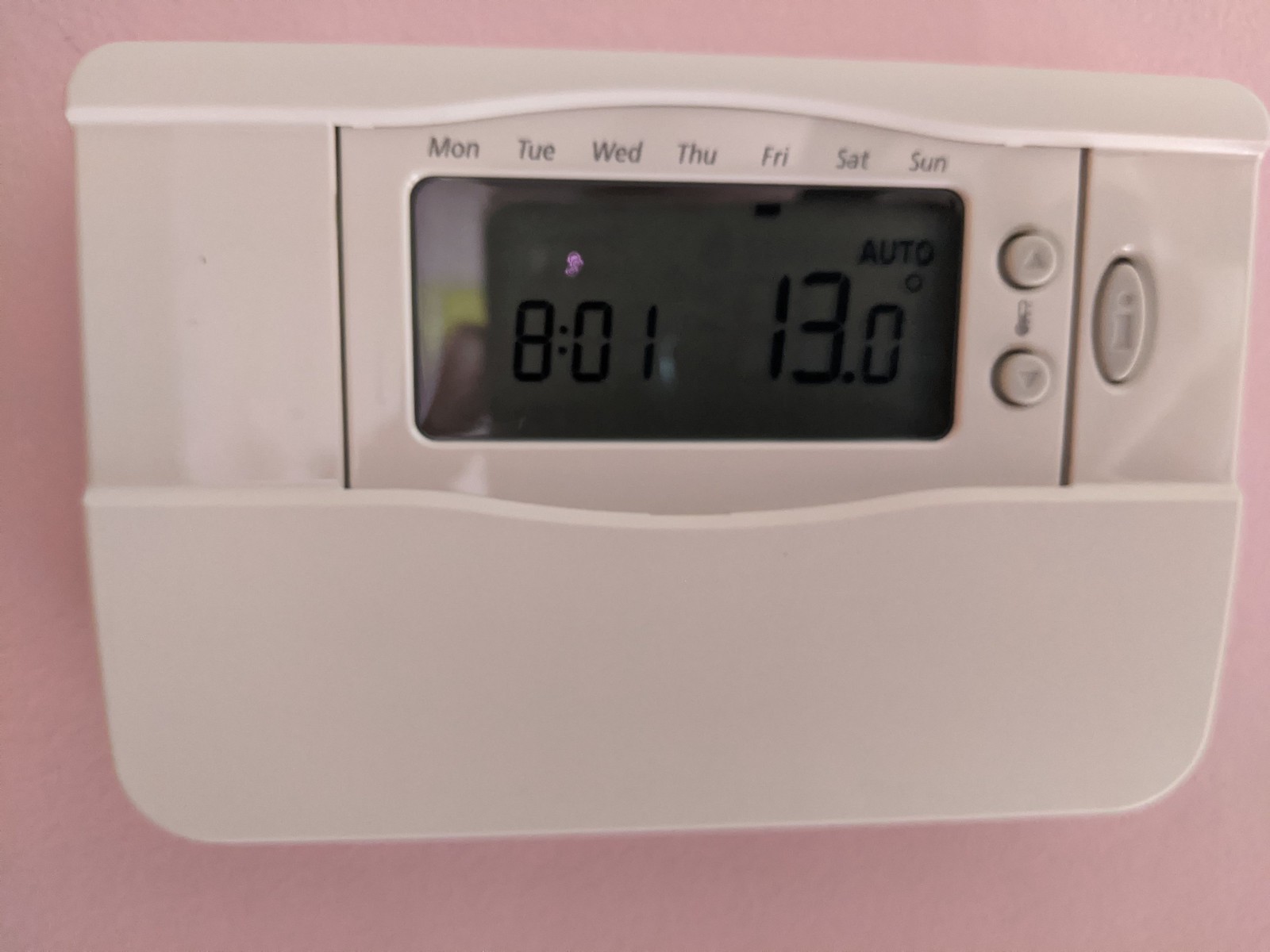This detailed image shows a white rectangular thermostat with rounded corners, mounted on a pink wall. The device’s screen occupies the top half, displaying the days of the week from Monday to Sunday (abbreviated as Mon, Tue, Wed, Thu, Fri, Sat, Sun), with a dot marking Friday. The time is indicated as 8:01, likely a.m., under the European 24-hour clock assumption. The temperature is set to 13.0 degrees Celsius and is currently in 'auto' mode. Beneath the display are temperature adjustment buttons with arrows for increasing and decreasing the temperature, and a menu button located below them. A small speck of pink paint is visible on the screen window of the thermostat.